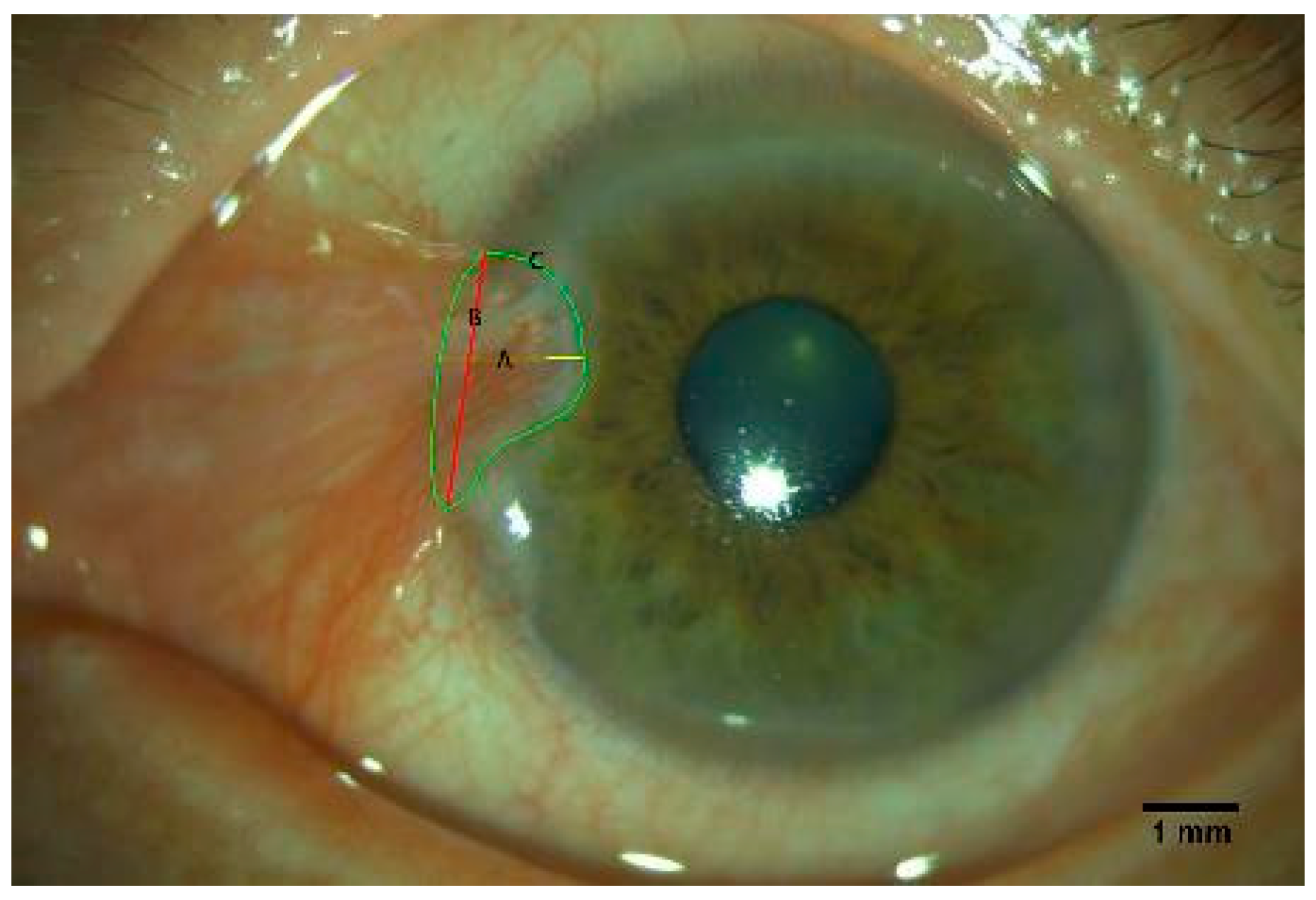This close-up photograph captures an eye in stunning detail, likely belonging to an animal given its unique coloration. The iris displays a vibrant mix of green and brown hues, and the central pupil appears almost black, with a noticeable reflection at the bottom. Surrounding the iris is the white sclera, interspersed with fine red blood vessels. A particularly prominent red area encroaches from the left side of the image, possibly indicating some abnormality or irritation. This section is also encircled by a slightly squiggly green line, labeled 'C'. A red vertical line labeled 'B' and a yellow horizontal line labeled 'A' correspond to specific areas on the eye. The image is scaled with a small black horizontal marker at the bottom right, labeled "1 mm" to indicate the magnification. Sparse eyelashes are visible at the top edges of the frame, further emphasizing the intimate proximity of the shot. The overall foggy and slightly blurred appearance suggests the presence of a vitreous fluid or another layer covering the eye.